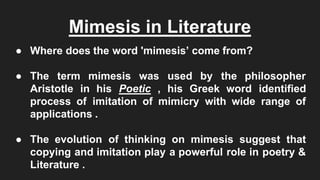The image features a horizontally-oriented slide designed for a college literature or English lecture. Against a black background, the slide prominently displays the title "Mimesis in Literature" in white letters, underlined for emphasis. Below this title, the content explains the term in three bullet points. First, it poses the question, "Where does the word mimesis come from?" followed by the explanation that "The term mimesis was used by the philosopher Aristotle in his Poetics. His Greek word identified a process of imitation or mimicry with a wide range of applications." Finally, the slide concludes by stating, "The evolution of thinking on mimesis suggests that copying and imitation play a powerful role in poetry and literature." This slide succinctly provides a detailed definition and historical context for the term "mimesis," tailored for educational purposes.